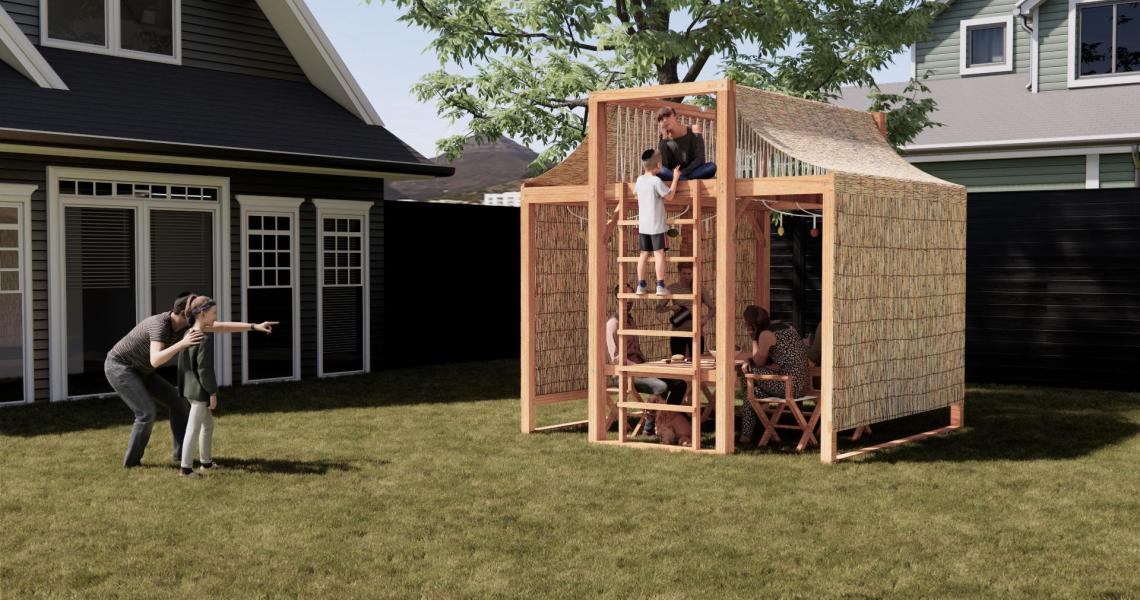The photograph captures a sunny afternoon in a backyard featuring a charming playhouse structure with a ladder. At the top of the structure, a little boy on the ladder gazes up at a girl who is seated. Below, three individuals are gathered around a table on the bottom floor of the playhouse. To the left, a father leans down, engaging in conversation and pointing towards the playhouse with his young daughter. Adjacent to them, a blue house with white trim and framed windows stands prominently. The scene is filled with shadows cast by the afternoon sun and a lush spread of grass.